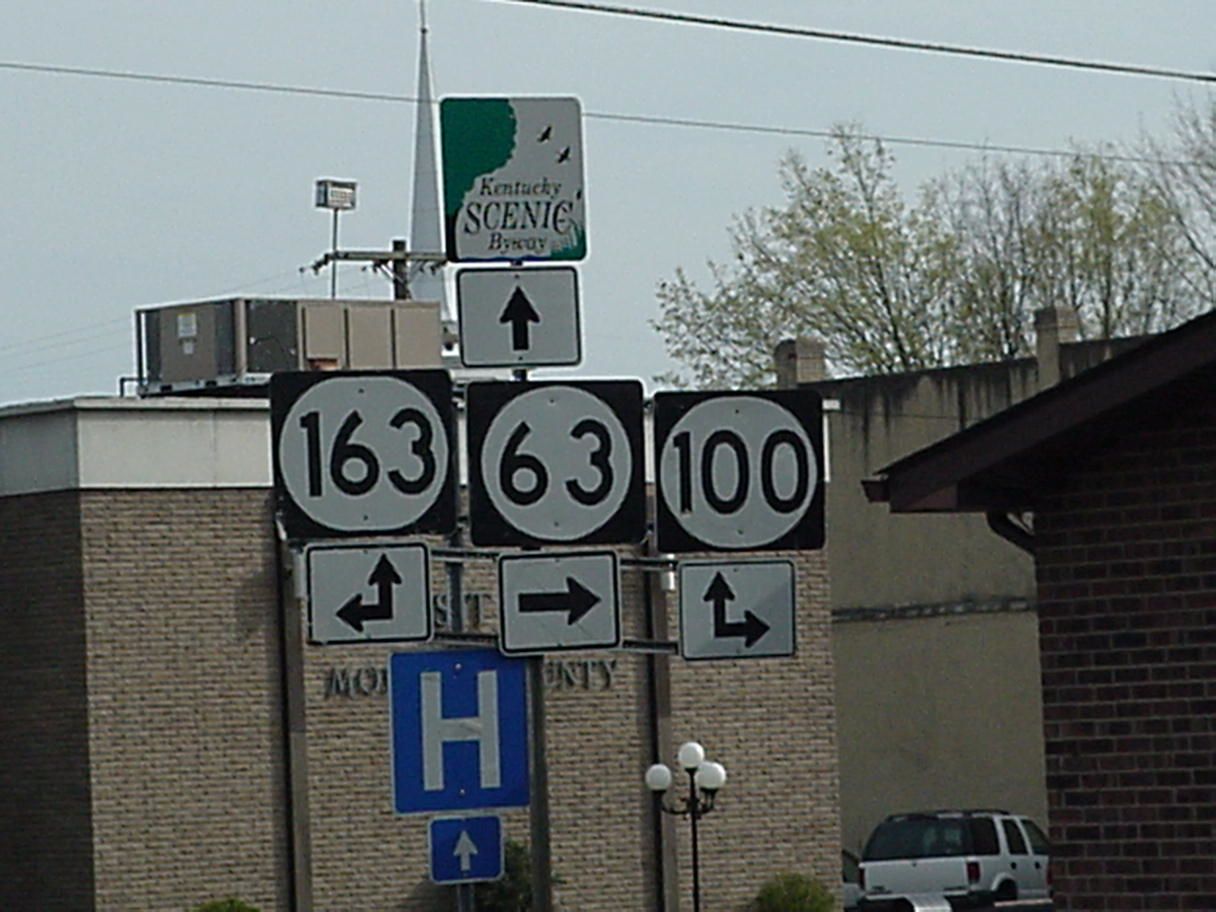A bustling street intersection is bathed in sunlight beneath a clear blue sky. Dominating the scene is a large, leafy tree stretching its branches over a series of buildings. To the left stands a robust brick building, and on the right, a smaller brick structure adds to the urban landscape. Adjacent to it, a substantial concrete building, in front of which a white car is parked, provides a contrasting texture. Prominently displayed at the center, a large directional sign reads "Kentucky Scenic" with route indicators: "163" in bold black letters on a white background outlined in black, "63" within a white circle surrounded by black, and "100" in black letters also on a white circle with a black border, each pointing towards different directions. Ahead, a blue hospital sign offers further navigational clues. Overseeing the intersection is a stately street light featuring three large, white spherical bulbs, adding a touch of elegance to the busy thoroughfare.